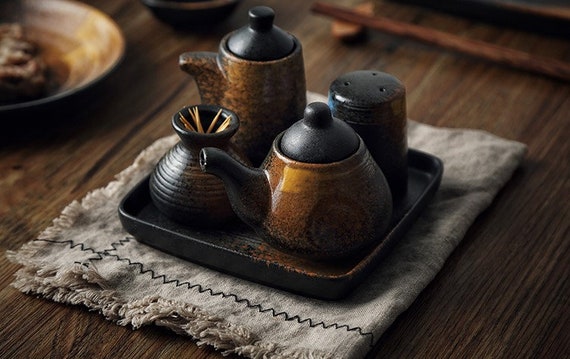The image showcases a detailed and realistic depiction of an antique Asian-inspired tea set, primarily crafted from dark brown and black ceramic materials, possibly porcelain. The tea set is elegantly arranged on a slightly distressed, blackened with hints of red, square tea tray. This tray is placed on a white, folded cloth adorned with black squiggly lines and a frilly edge, all atop a dark wooden table.

At the center of the composition, there's a prominent teapot with a reddish-brown body and a black lid. To its left is a distinctive V-shaped container, colored in black with ridges, holding tan stirring sticks or perhaps toothpicks. Another vessel, resembling a creamer container, sits behind the teapot, featuring similar colors and a design suggestive of liquid storage. To the right of the teapot is a cylindrical shaker, likely used for condiments like salt, identifiable by its black color and three holes on top. The set includes various other items, such as a round plate with contents on the left and possibly another bowl to the right, adding to the intricate assembly of this historic, aesthetically pleasing tea set.